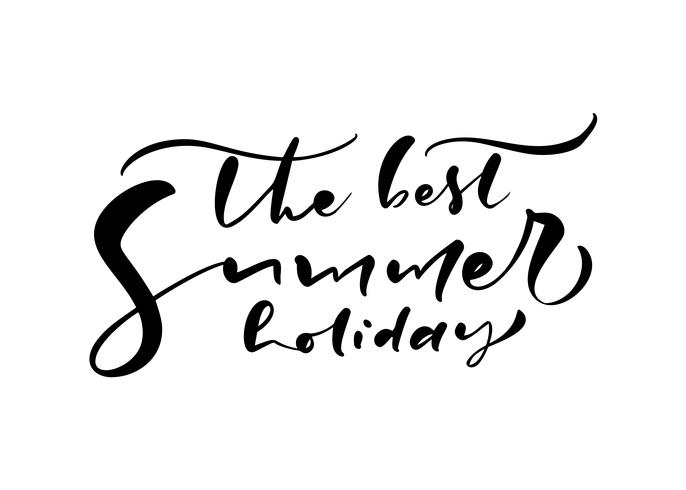The image features highly stylized, black, curvy text on a white rectangular background that reads, "The best summer holiday." The text is arranged with "The" and "best" on the top row, "summer" prominently in the middle, and "holiday" at the bottom. The letter "S" in "summer" is exceptionally large, taking up almost a quarter of the image on the left side. The T's in "the" and "best" have exaggerated, wavy tops that extend across the words, giving them an undulating, wave-like appearance. The R in "summer" is also disproportionately large compared to the surrounding letters. The overall design is reminiscent of calligraphy or computer-generated stylization, lending an elegant and eye-catching effect. This text layout and styling suggest it could be used as a logo, possibly for a greeting card, an invitation, or an advertisement related to a summer sale or event.